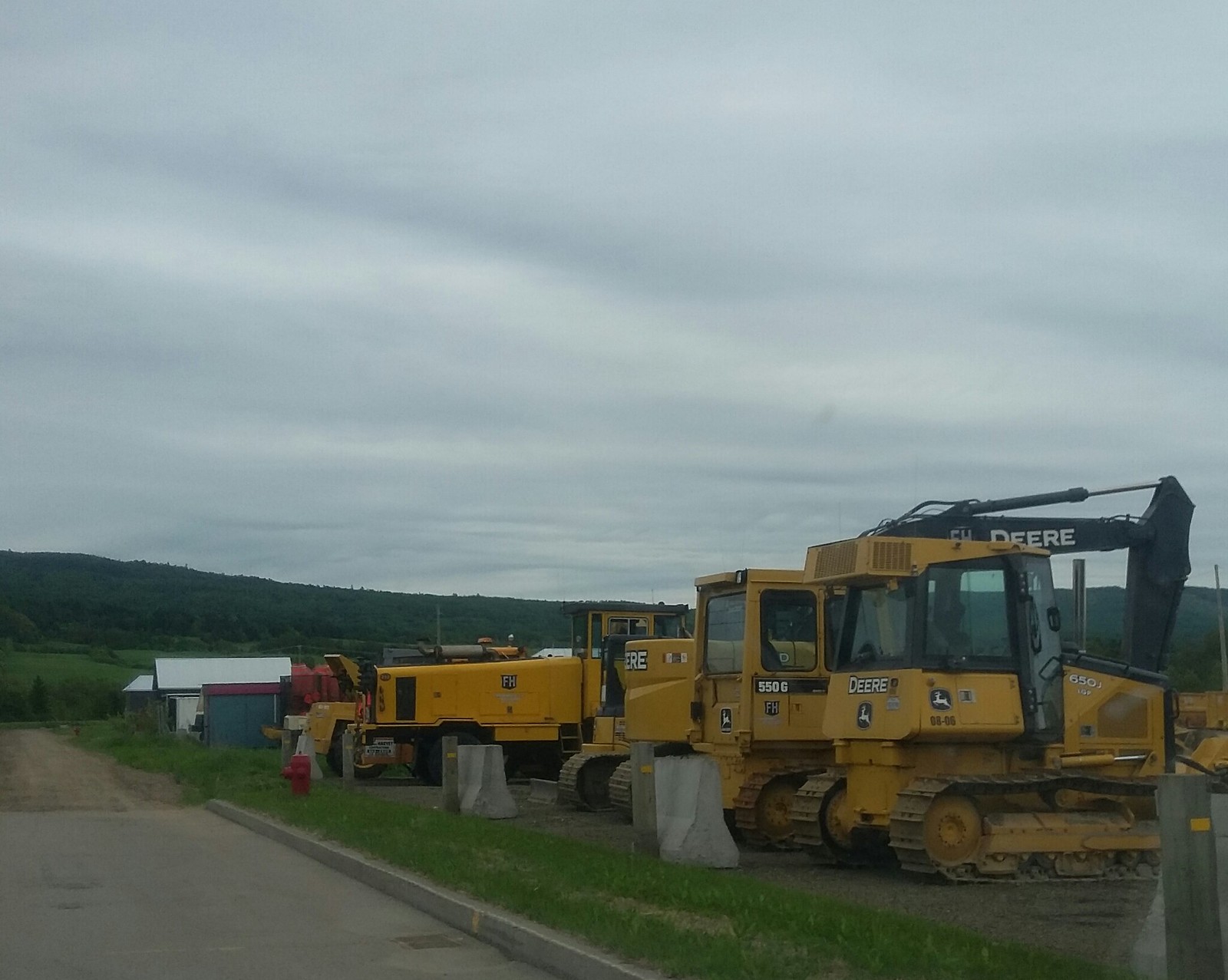This color photograph, slightly wider than vertical, captures a collection of John Deere yellow construction machines parked on a grassy field adjoining a road. The image was taken on an overcast day under a gray sky, indicative of recent rainfall. The far-reaching field is complemented by rolling hills visible in the distance. Each vehicle prominently displays the John Deere logo, featuring a green crest with a leaping deer, and some machines bear the text "550G" along with the brand name "Deere" in bold white letters with black outlines. The equipment includes a range of machinery, such as a digging shovel and a tractor-like vehicle fitted with a large plow. Additionally, a large black hydraulic crane extending from one vehicle is clearly marked with the "Deere" name. The vehicles, parked next to each other, stand out against the gently undulating landscape, which also includes a few sheds nearby.